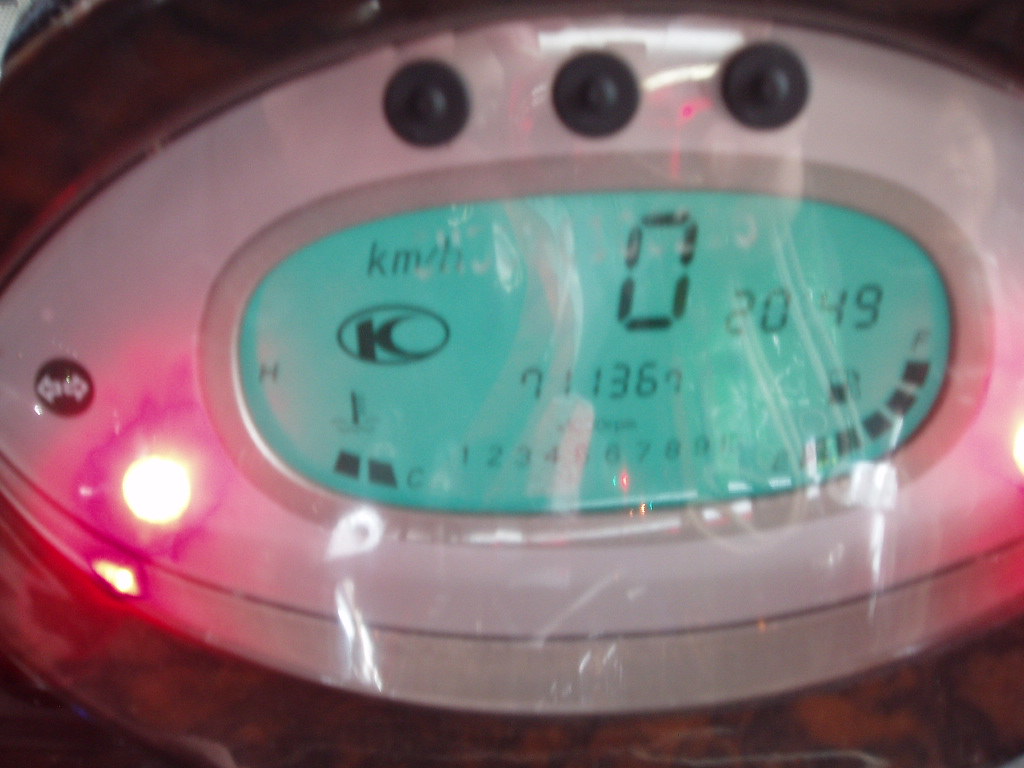This image features a digital clock with a display showing the time as "0:00" and the year "2049" next to it. The screen has a blue background and appears to be covered by a layer of clear plastic wrap. Positioned above the display are three buttons, and to the left, a red light is flashing. Below the "0:00" time display, there are additional numbers: "711367". Overall, the device seems encased in a translucent, protective plastic covering.